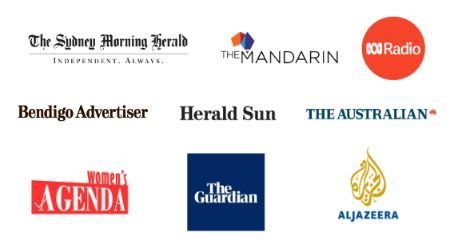The image showcases nine distinct newspaper logos displayed prominently against a clean white background. These logos are meticulously arranged in a grid format, consisting of three rows and three columns. 

In the topmost row, from left to right, are the logos for the Sydney Morning Herald, the Mandarin, and a radio logo characterized by its text enclosed within an orange circle. 

The middle row features, beginning from the left, the logo for the Bendigo Advertiser, followed by the Herald Sun, and then the Australian, which is presented in blue text.

The final row at the bottom displays, from left to right, the Women's Agenda logo in a striking combination of orange and white, next to the Guardian's logo set within a dark square background, and finally the Al Jazeera logo, elegantly rendered in blue and gold, positioned in the lower right corner.